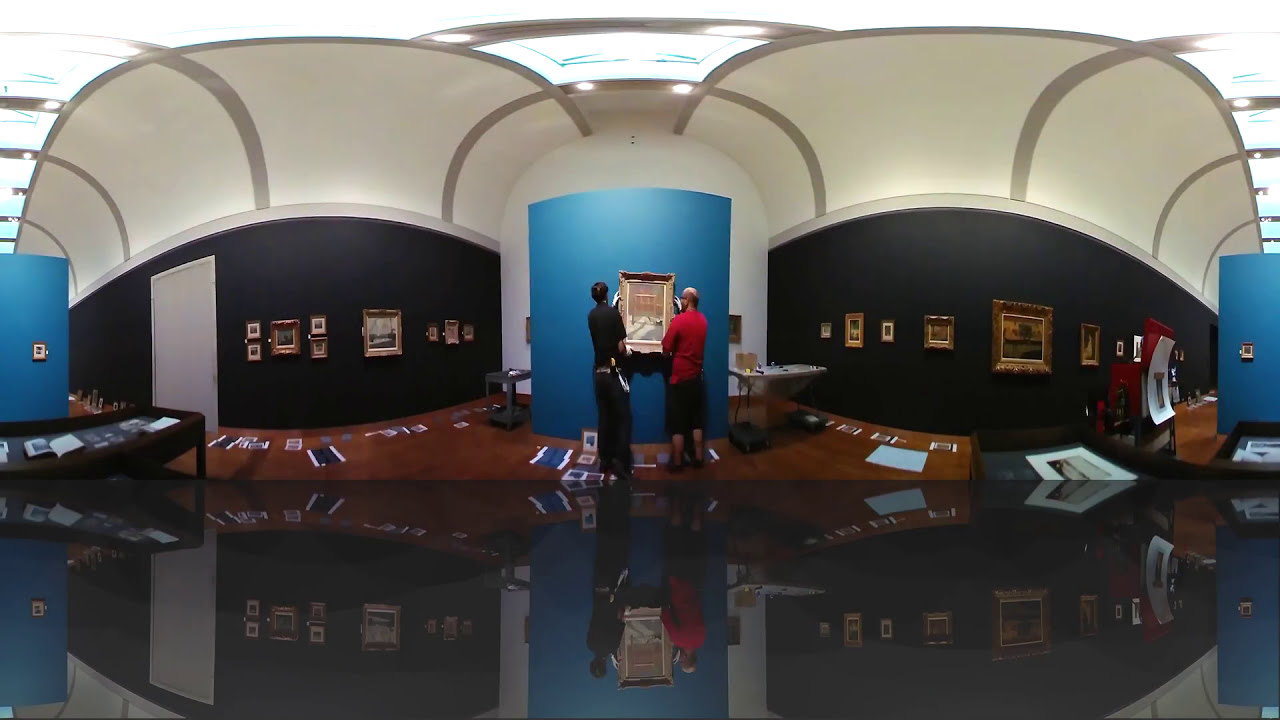This image is a highly detailed, panoramic view of a large art gallery, captured using 360 imaging, which results in some noticeable warping, especially at the ceiling and edges. The gallery is rectangular and horizontally oriented, featuring extensive skylights that flood the space with natural light. The gallery walls are an intricate interplay of colors and designs: the left and right walls feature a striking half black, half white theme, with a curved white arch ascending towards the ceiling, adorned with gray, silvery metal stripes placed about six feet apart. These stripes enhance the sense of depth and space by curving upward and outward.

At the lower portion of these arches, a dark, dark blue band runs horizontally, covered with rows of framed artworks. Centrally placed within the gallery is a notable blue vertical rectangle adjacent to a light blue vertical rectangle, both serving as a backdrop for a large, framed painting that appears to depict a building. Two men are intently focused on this particular piece; the man on the left is dressed in black, while the man on the right wears a red top with black shorts. They are either observing or potentially hanging the artwork, engrossed in their task.

Throughout the gallery, additional framed artworks decorate the gray walls, which flank a doorway on one side. The blue sections of the walls, appearing on both the left and right, are actually the same due to the panoramic nature of the image. The overall design and artifacts give the impression of an educational space, possibly an art studio within a college, emphasizing both the creative and academic ambiance of the setting.